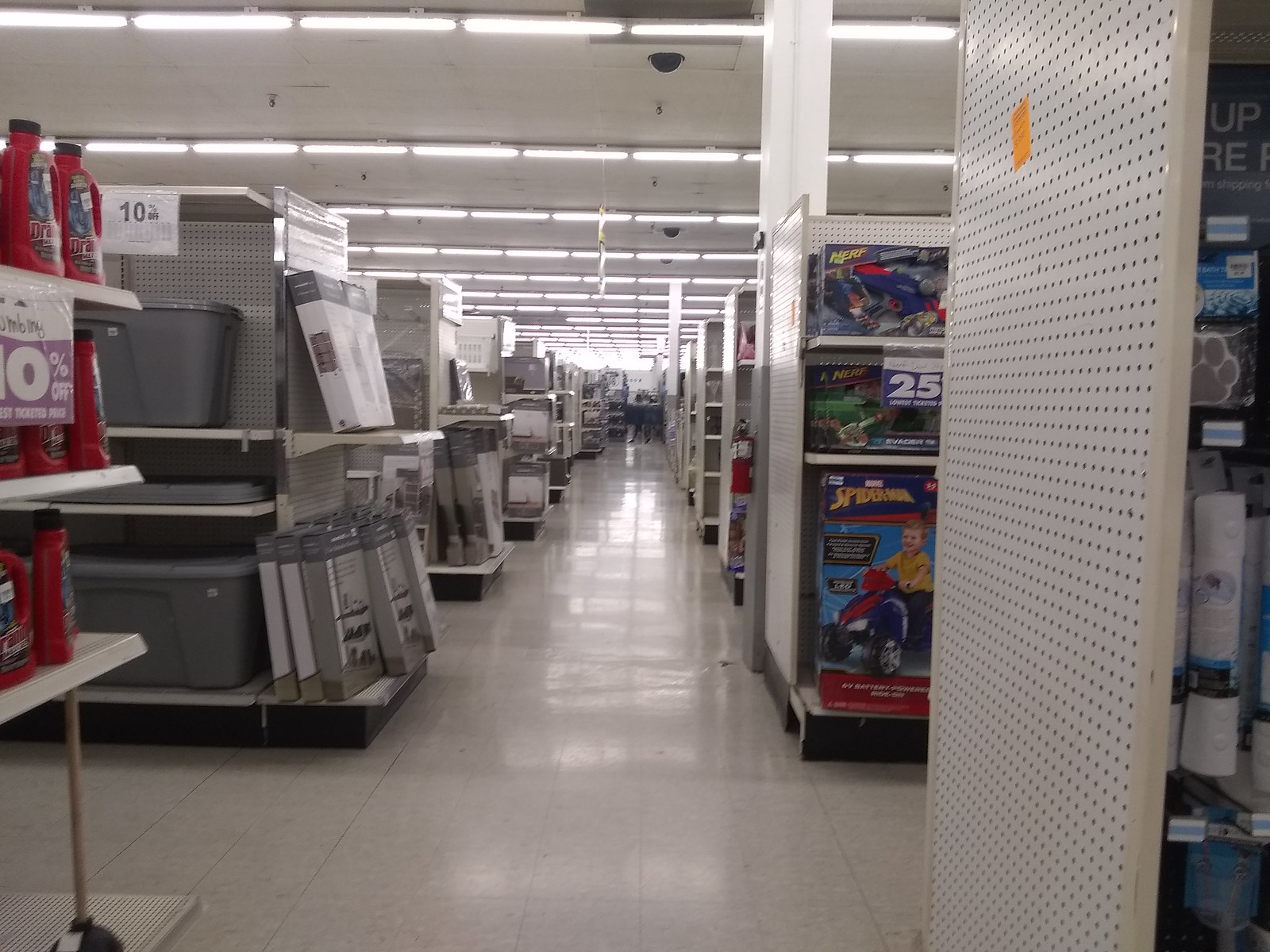The image portrays a typical American retail store, likely a Walmart or Target, situated in the home and toy aisles. The shelves appear partially stocked, indicative of ongoing inventory adjustments. In the foreground, a promotional display features drain cleaners and plungers, advertised at a discounted rate of 40% off. To the right, the toy aisle showcases items with a 25% discount, suggesting efforts to clear out inventory during a reorganization. Overhead, fluorescent lighting illuminates the scene, common to such retail environments. A security camera, strategically placed to monitor every other aisle, hints at standard anti-theft measures. The overall atmosphere reflects a commonplace American shopping experience, characterized by routine store layouts and inventory management practices.